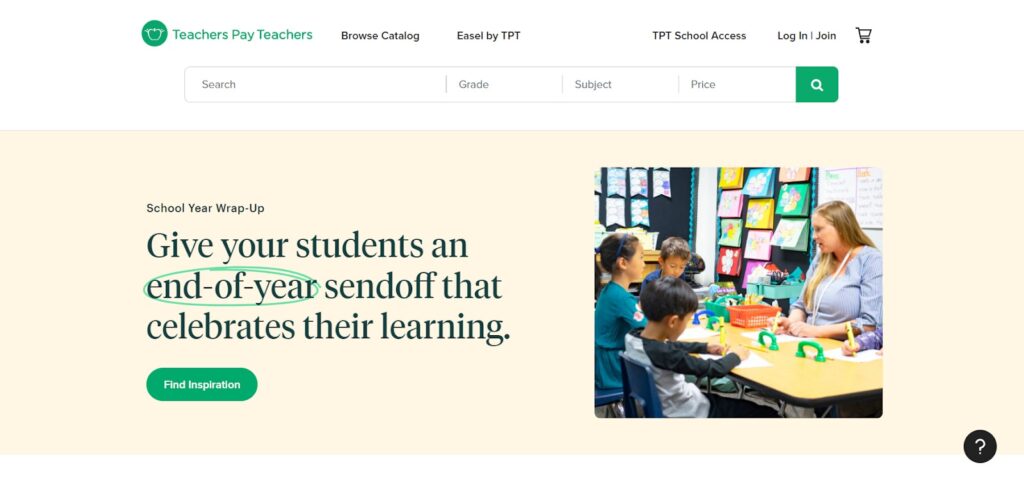The webpage displayed features a clean, white background with a green icon at the top that includes a small apple graphic and the text "Teachers Pay Teachers" in green. Adjacent to this icon, several options are listed in black text: "Browse Catalog," "Easel by TPT," "TPT School Access," and "Login | Join." A shopping cart icon is positioned at the far right of this top navigation bar.

Beneath this, a large search bar spans the width of the page, offering the options to search by grade, subject, and price, separated by vertical bars. A green search button with a search icon is located on the right-hand side of the search bar.

Directly below the search bar, a full-page width horizontal rectangle features a yellowish-tan background. This section is split into two parts. On the right-hand side, there is an image of a teacher with three students in a classroom setting. To the left, bold text reads "School Year Wrap-Up," alongside a message encouraging teachers to give their students an end-of-year send-off that celebrates their learning. The phrase "End of year" is circled in green. Beneath this text, a green oval button with white text reads "Find Inspiration."